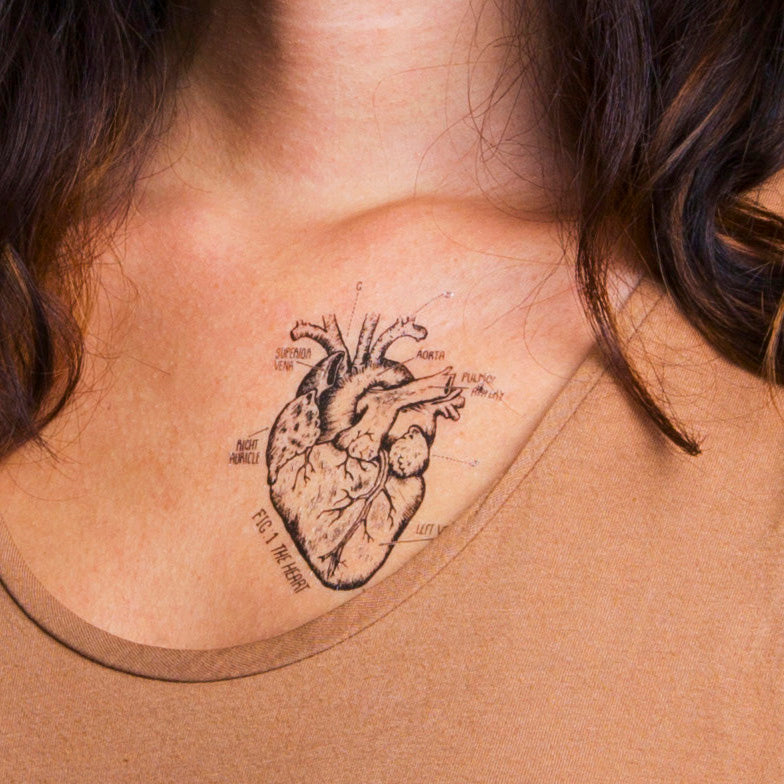In this detailed image, a woman with shoulder-length brown hair interspersed with lighter highlights is wearing a light tan, low-cut shirt. Prominently displayed on the upper part of her chest, near her collarbone, is a meticulously detailed black and gray tattoo of a human heart. The tattoo, featuring precise anatomical details, showcases labels including the "aorta" at the top and the "left ventricle" toward the bottom. Additionally, there are dotted lines and labels pointing to various parts of the heart. Beneath the heart, the tattoo includes the text "FIG.1: The Heart," further emphasizing its instructional design. The woman's face is not visible; the focus remains on the intricate heart tattoo and its anatomical annotations.